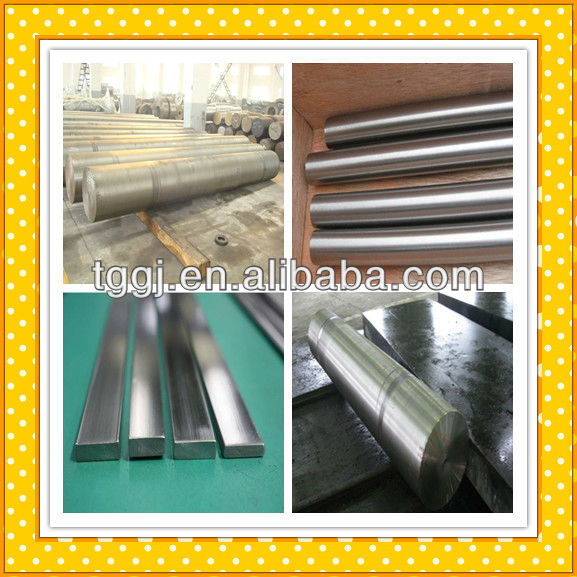The image depicts a digitally-created frame with a gold border adorned with white polka dots and encasing four smaller photos in a window pane style format. Each photograph showcases different metal objects, systematically arranged for an industrial advertisement, potentially on Alibaba, as indicated by the text "TGGJ.en.alibaba.com."

In the upper left, there's a large, heavy-looking cylindrical metal object. To its right, another cylinder appears, smaller and shinier compared to the first. The bottom left panel features four long rectangular metal bars placed on a green platform, resembling silver Kit Kat bars. Lastly, the bottom right panel displays another cylindrical metal rod on what seems to be black boxes.

The color palette within the frame includes shades of orange, black, yellow, white, gray, silver, turquoise, and brown, contributing to the industrial vibe of the presentation. Each metal object is meticulously positioned, providing a clear and detailed overview suitable for showcasing different metal products.